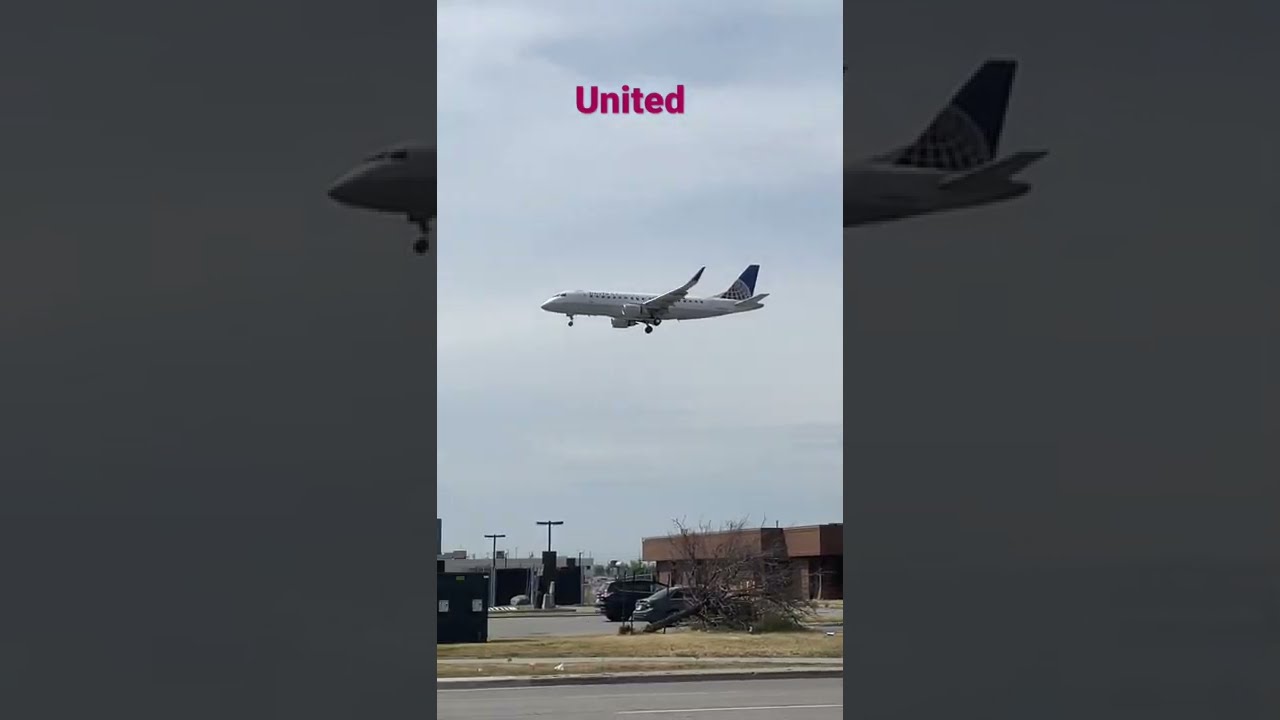This image, likely captured with a mobile phone and oriented vertically, depicts a landing jumbo jet branded with the word "UNITED" in a magenta serif font across the top. The aircraft, which resembles a United Airlines plane with a distinctive blue fin and insignia on the tail, is flying low over a town. Below, the scenery includes a brown brick building, a parking lot with a couple of parked cars, overgrown grassy areas, and sidewalks. There are noticeable details like a spindly, dead tree lying sideways on the ground, indicative of a neglected area. The sky above is overcast with gray clouds, adding to the somber, fall-like atmosphere of the scene.